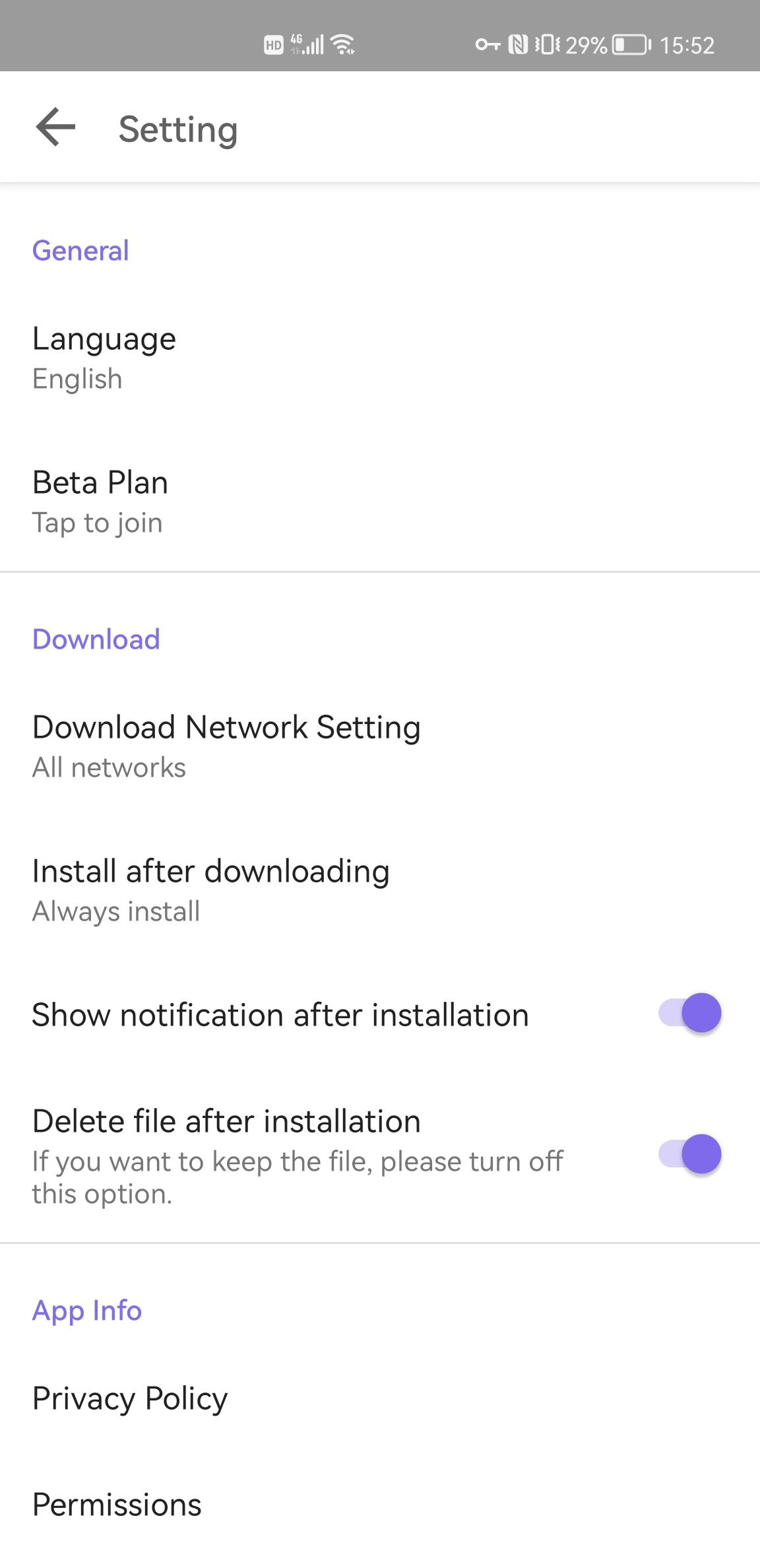This mobile screenshot captures the settings screen of an application, rendered primarily in medium gray with black text, gray subtext, and vibrant purple accents highlighting headers and toggles. At the very top of the screen, "Settings" is displayed in black with a left-pointing arrow beside it. Below, sections are clearly segmented with purple headers. The first section title, "General," is in purple, beneath which are options like "Language" displayed as "English," and "Beta Plan" with the subtext "Tap to join."

The next segment, titled "Download" in purple, focuses on download preferences. Under this, "Download Network Settings" is listed in black text with the subtext "All Networks" in gray. Additional options include "Install After Downloading" in black, and beneath it "Always Install" in gray. A notable feature, "Show Notification After Installation," has a purple toggle that is switched on. Similarly, "Delete File After Installation" also has its purple toggle activated, accompanied by a gray subtext cautioning, "If you want to keep the file, please turn off this option."

Towards the bottom, the purple header "App Info" leads to options such as "Privacy Policy" and "Permissions," both in black text. At the very top of the screen, standard status icons are visible for battery, time, Wi-Fi, and signal strength, providing essential device information.